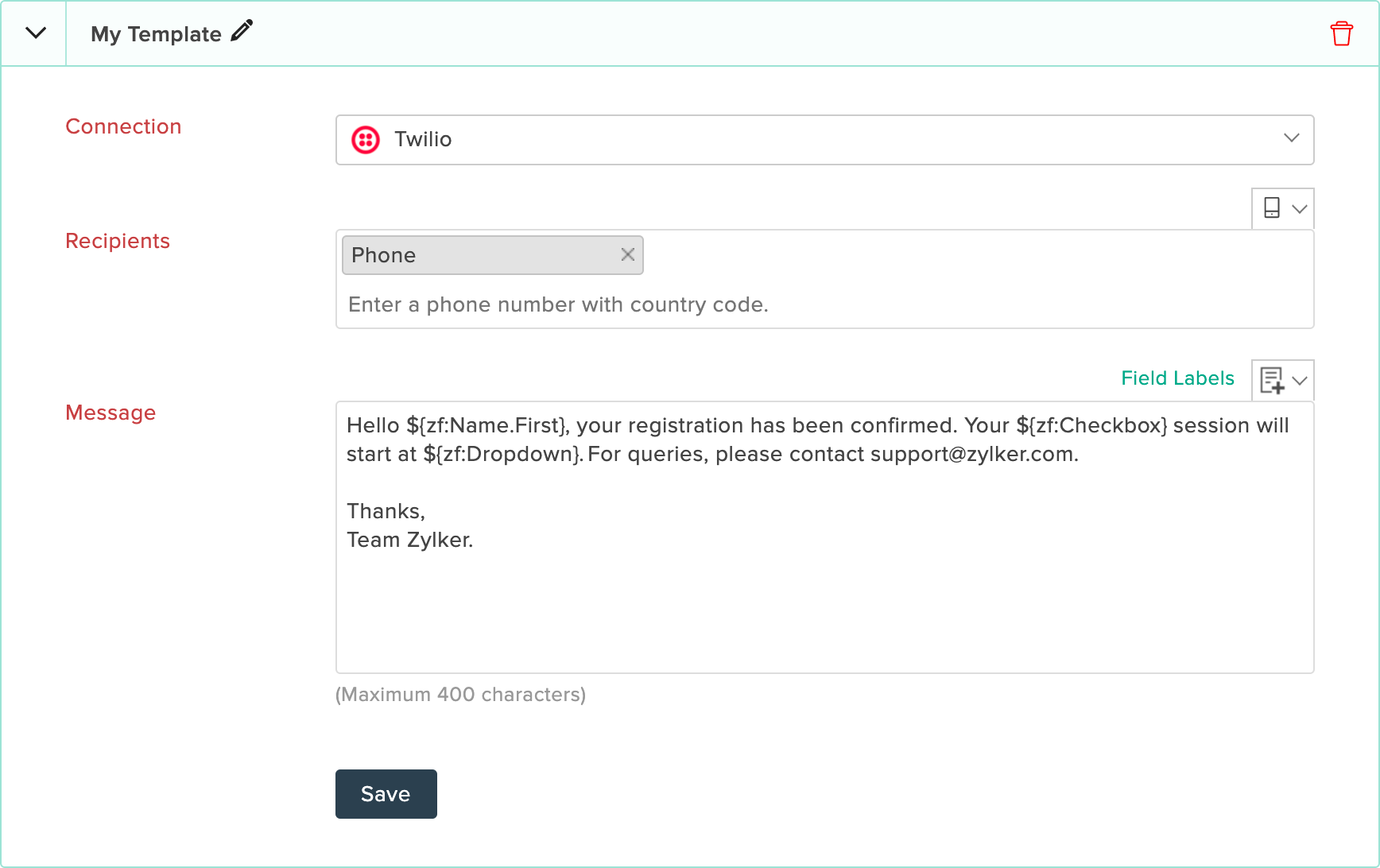This image is a screenshot of an email template editor interface with a clean white background. In the upper left-hand corner, there's a dropdown arrow next to the words "My Template" and an adjacent pencil icon. The upper right-hand corner displays a trash can symbol, indicating the option to delete the template.

On the left side of the screen, there are three labeled sections in red text: 

1. **Connection** 
2. **Recipients**
3. **Message**

Next to the "Connection" label, there is a dropdown box with "Twilio" selected.

Under the "Recipients" section, there is a text box labeled "Phone" with instructions below it that read, "Enter a phone number with country code."

In the "Message" section, the composed text reads:
"Hello $ZF:name.first,  
Your registration has been confirmed.  
Your $ZF:checkbox session will start at $ZF:dropdown.  

For queries, please contact support at zylker.com.

Thanks,  
Team Zylker"

Below the message, there is a note indicating, "Maximum 400 characters," and a button labeled "Save" is available to save the current template.